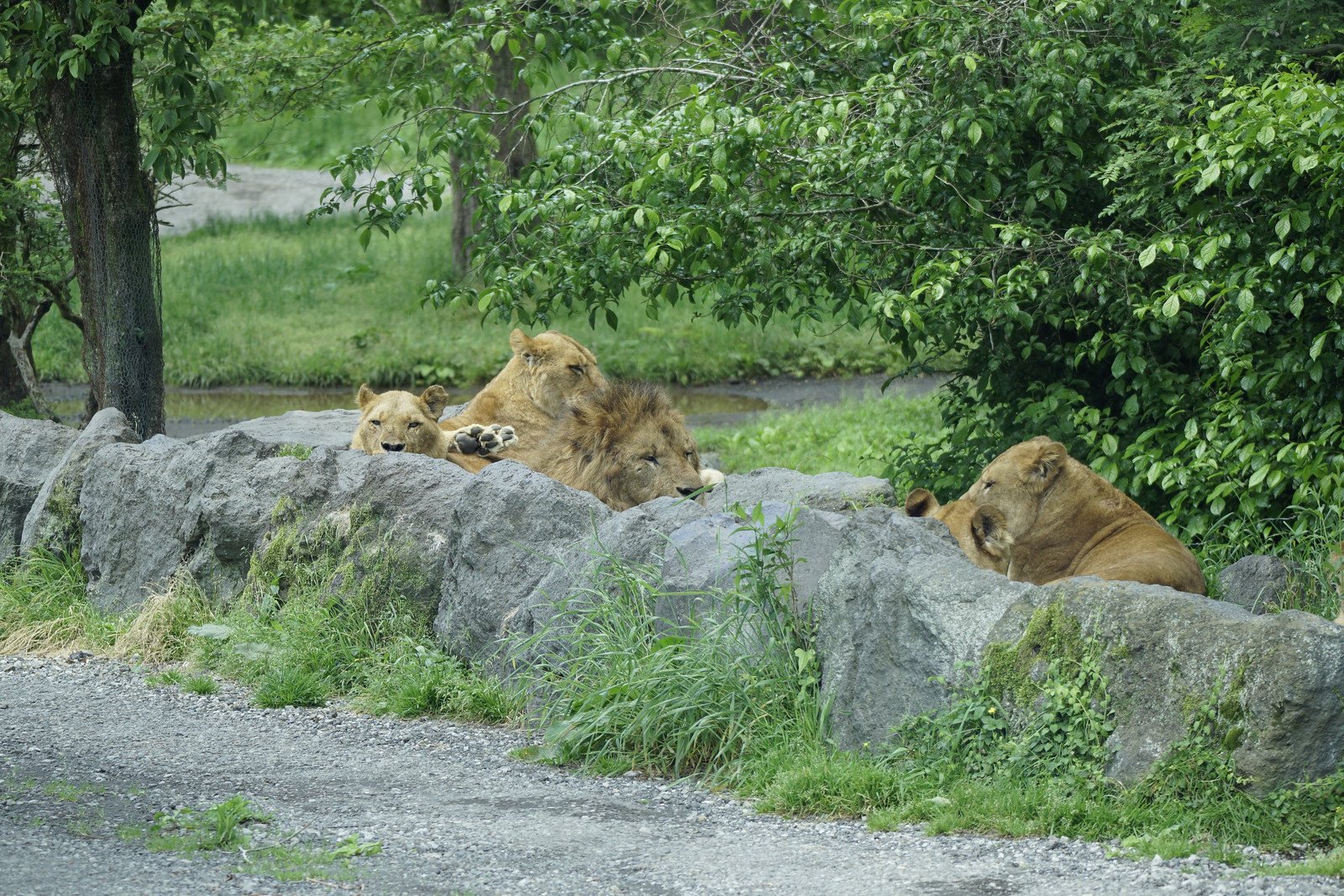This detailed photograph captures a group of lions resting in what appears to be a safari park or zoo, as the setting is a green woodland rather than the typical plains. The scene showcases a gravel roadway in the foreground, bordered by a small stretch of grass that leads to a low-level wall made of gray rocks, some of which are adorned with green moss. Just behind these rocks, the lions are lounging. Prominently in the middle is a majestic male lion with a noticeable mane, flanked by three lionesses; two are positioned slightly behind him, and a third is lying facing him. In the distance, a small creek can be glimpsed, bordered by lush bushes and trees with low-hanging green branches. The entire area is surrounded by verdant foliage, enhancing the tranquil ambiance of the scene. The roadway curves around, adding depth to the image and suggesting a natural extension of the habitat.